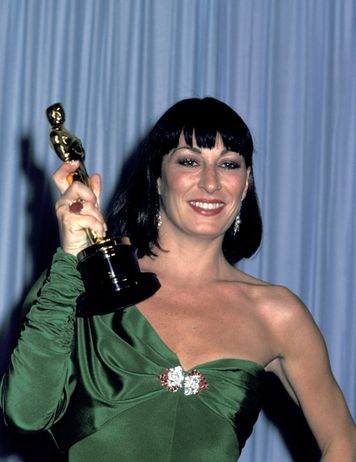The color photograph captures a famous white actress, possibly named Angela, with a radiant smile. She has shoulder-length black hair featuring blunt cut short bangs and is adorned in long silver earrings. Her attire is a stunning green satin or silk dress; it has a unique asymmetrical design with one sleeve and a sleeveless sweetheart neckline on the other side. The dress is backless and embellished with a pink and diamond brooch at the chest, adding to its elegance. In her right hand, she proudly holds up an Oscar statuette, positioning it to the right of her head and slightly forward, her bejeweled red ring visible on her right ring finger. Her left hand is not visible. The striking blue curtains in the background contrast sharply with her dress, and she casts a shadow on them, accentuating the image's depth. The image is bathed in bright, natural light, highlighting every detail and capturing the moment's essence vividly.